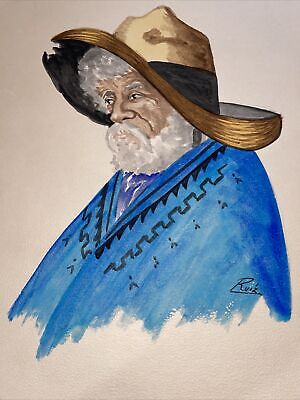This artwork is a watercolor illustration on an aged, tan, and slightly faded paper. It portrays an older gentleman with dark skin, featuring striking white hair and a full white beard that give him a Santa Claus-like appearance. He is adorned in a wide-brimmed brown cowboy hat, which has a distinctive black stripe near its bottom and a broken front edge. The man is clad in a layered poncho that transitions from light blue to dark blue, accented with black stripes or trim around the collar. The portrait captures him staring to the left, and it ends midway down his chest, giving it an unfinished yet textured look. The background of the painting is a light beige, enhancing the central figure. In the bottom right corner of the poncho, there is the artist's signature, "Ruiz."